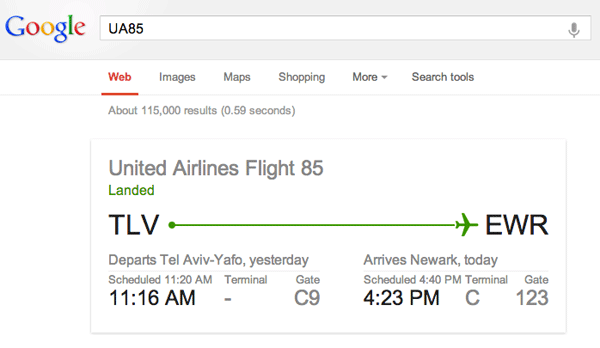The Google search results page is displayed prominently, with the classic Google logo at the top left, featuring the familiar blue, red, yellow, and green colors. Just below the logo is the search bar, containing the query "UA85." Underneath the search bar, there are options for different types of searches: web, images, maps, shopping, and more. The web option is selected and highlighted in red, while the others remain in gray. 

The search results indicate approximately 115,000 results found in 0.59 seconds. A key result stands out, providing detailed information about United Airlines flight UA85. The information is bordered by a light gray line, distinguishing it from the rest of the page content. 

The flight details include:
- Flight Number: UA85
- Status: Landed in Tel Aviv (TLV)
- Departure: Newark Liberty International Airport (EWR)
- Departure Date: The previous day
- Scheduled Departure Time: 11:20 AM
- Actual Departure Time: 11:16 AM
- Departure Terminal: C
- Departure Gate: C7
- Arrival Date: Today
- Scheduled Arrival Time: 4:40 PM
- Actual Arrival Time: 4:23 PM
- Arrival Terminal: C
- Arrival Gate: 12, 3

An airplane icon is displayed on the right side, along with a green line indicating a successful status. The page features a mix of colors, including blue, red, yellow, green, gray, black, and white.